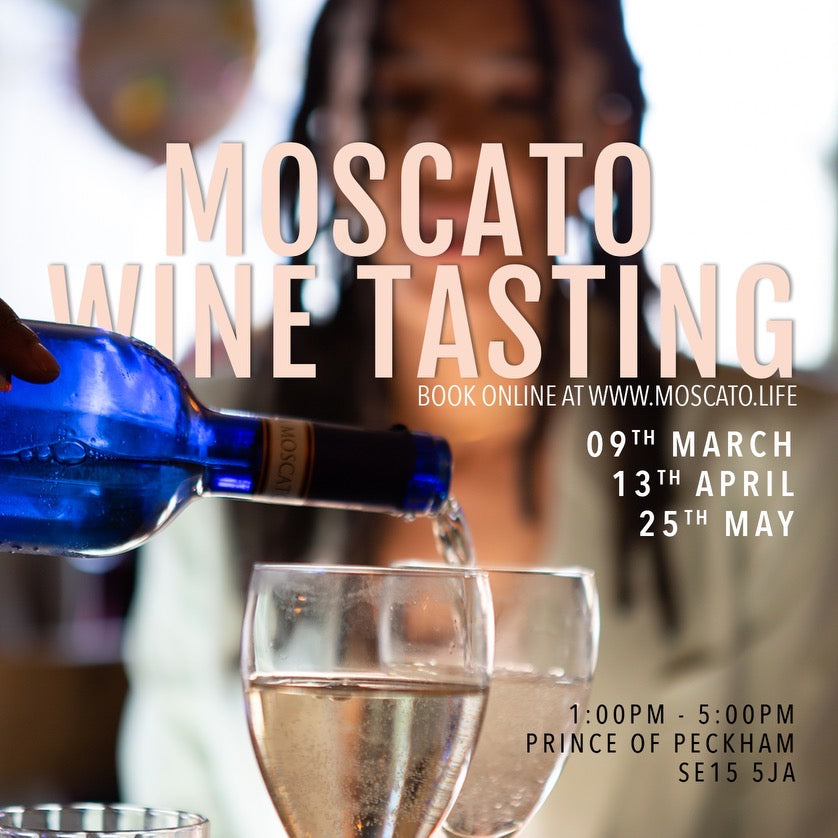This advertisement for a Moscato wine tasting event prominently features the headline "MOSCATO WINE TASTING" in large, peach-colored block letters slightly above the center of the image. Below this headline, in smaller peach text, reads, "book online at www.moscato.life." Aligned with the right margin, you'll find a list of dates in white text: "09-March, 13-April, 25-May," followed by event details in black text: "1-5 PM, Prince of Peckham, SE15 5JA."

The background of the advertisement showcases a young woman with dark hair styled in braids or dreads, wearing a light-colored open-cut long-sleeve shirt, though she remains blurred. There is also a pink balloon with a yellow circle behind her, adding a festive touch. The foreground, in sharp focus, captures a person with darker skin pouring Moscato from a striking sapphire-blue bottle into one of two wine glasses, which are nearly three-fourths full. This creates a vivid contrast emphasizing the act of pouring and the sparkling clear liquid of the Moscato wine.